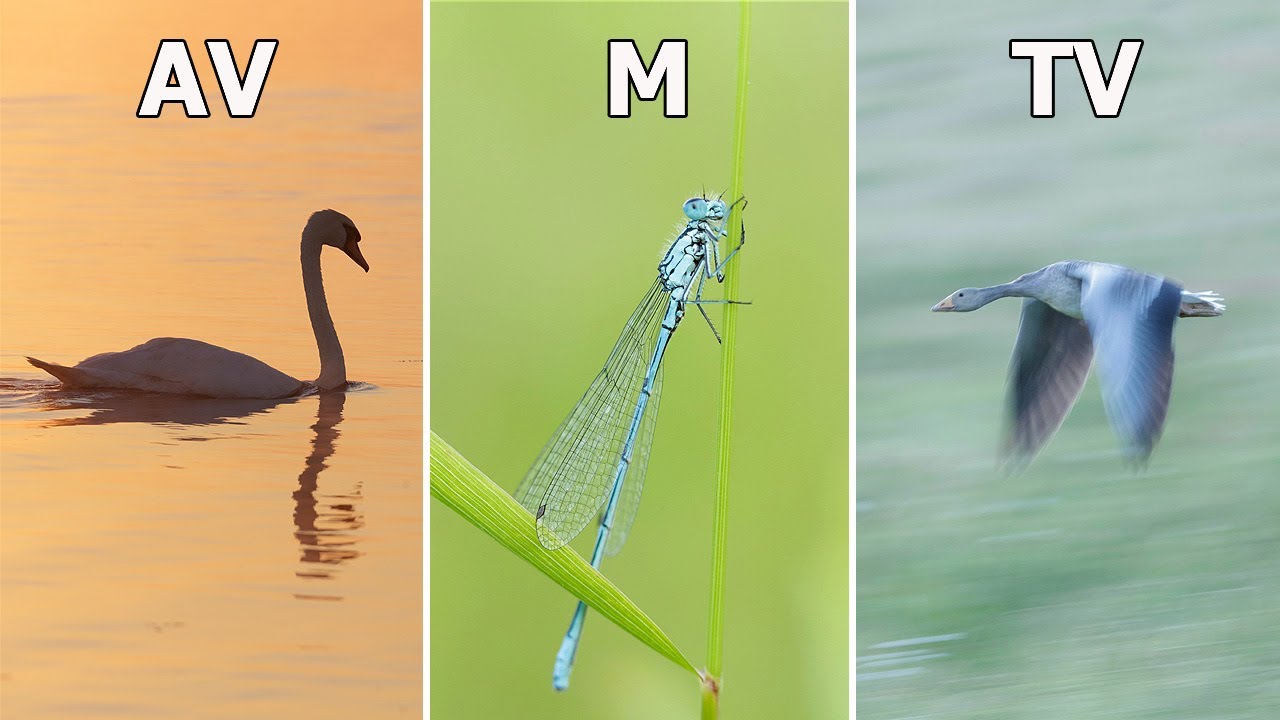The image is a collage of three detailed photographs demonstrating wildlife photography. On the left side, the top picture features a balding man with glasses and dark hair, dressed in a blue jacket. He is holding a black camera with a large zoom lens, standing against a wire fence with dense brown brush behind him. Below this is a close-up of the same camera, showing the man's hand adjusting the aperture of the lens. The camera is resting on a wooden fence post, with green grass visible beneath. On the right side of the collage is an exquisite picture of a male bullfinch perched on a branch adorned with flowery leaves. The bird has a striking orange breast, gray and black wings, a black head and beak, and a white underbelly, set against a yellow-brown blurred background. The sequence captures the process of photographing a beautiful wild bird.